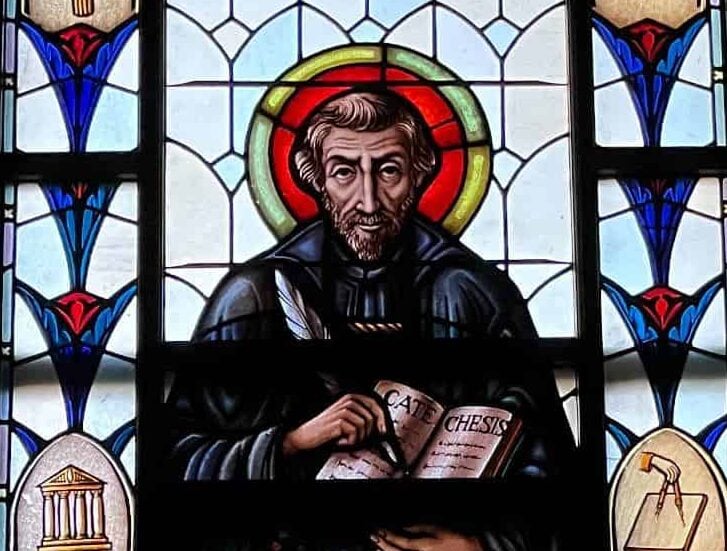This photograph depicts a vibrant and colorful stained glass window in a church setting, showcasing an intricately detailed central figure, likely a saint. The central figure, with shoulder-length brown hair swept back, a beard, mustache, and expressive dark eyes, gazes directly at the viewer. His forehead and eyes are lined with wrinkles, and he possesses a substantial nose. A radiant halo encircles his head, featuring an outer rim of yellow and green and an inner red ring close to his head. This figure is clad in a navy blue cloak, holding a book outward with "Kate Chasis" (or "Catechism") inscribed on its cover and a quill pen poised against the book in his other hand. 

Flanking the saint are intricate arched designs incorporating elaborate leading that segment the stained glass into various shapes. On the right side, a hand holding a compass over a piece of paper is depicted, while the left side features a columned building resembling classical architecture. The decorative glass columns on either side are predominantly blue, ascending into floral-like designs with red triangular accents at the top, enhancing the window's overall aesthetic richness.